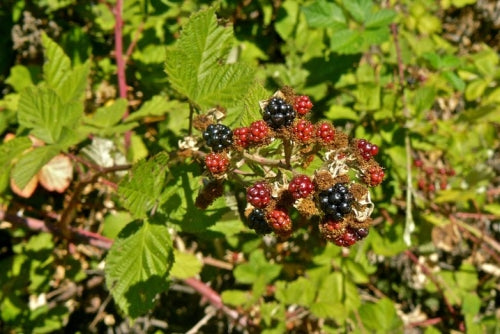This close-up, overhead daylight photograph captures a vibrant cluster of blackberries and immature red berries, nestled within a wooded brush area. The berries are the focal point, positioned centrally amidst bright green leaves with a striking mix of colors. The blackberries, approximately five in number, exhibit a deep, glossy black while the younger, smaller red berries – possibly unripe blackberries – add vivid contrast. Scattered around the main cluster, you can spot additional red berries and various plant stems and leaves, creating a lush, but slightly blurred backdrop. The sun appears to shine down from the top left, casting a gleam on the berries and illuminating a red stick that juts out from among the foliage. The combination of sharp and softer elements, marked by interplays of light and shadow, gives the scene a rich, textured feel, capturing a moment in nature’s growth process.